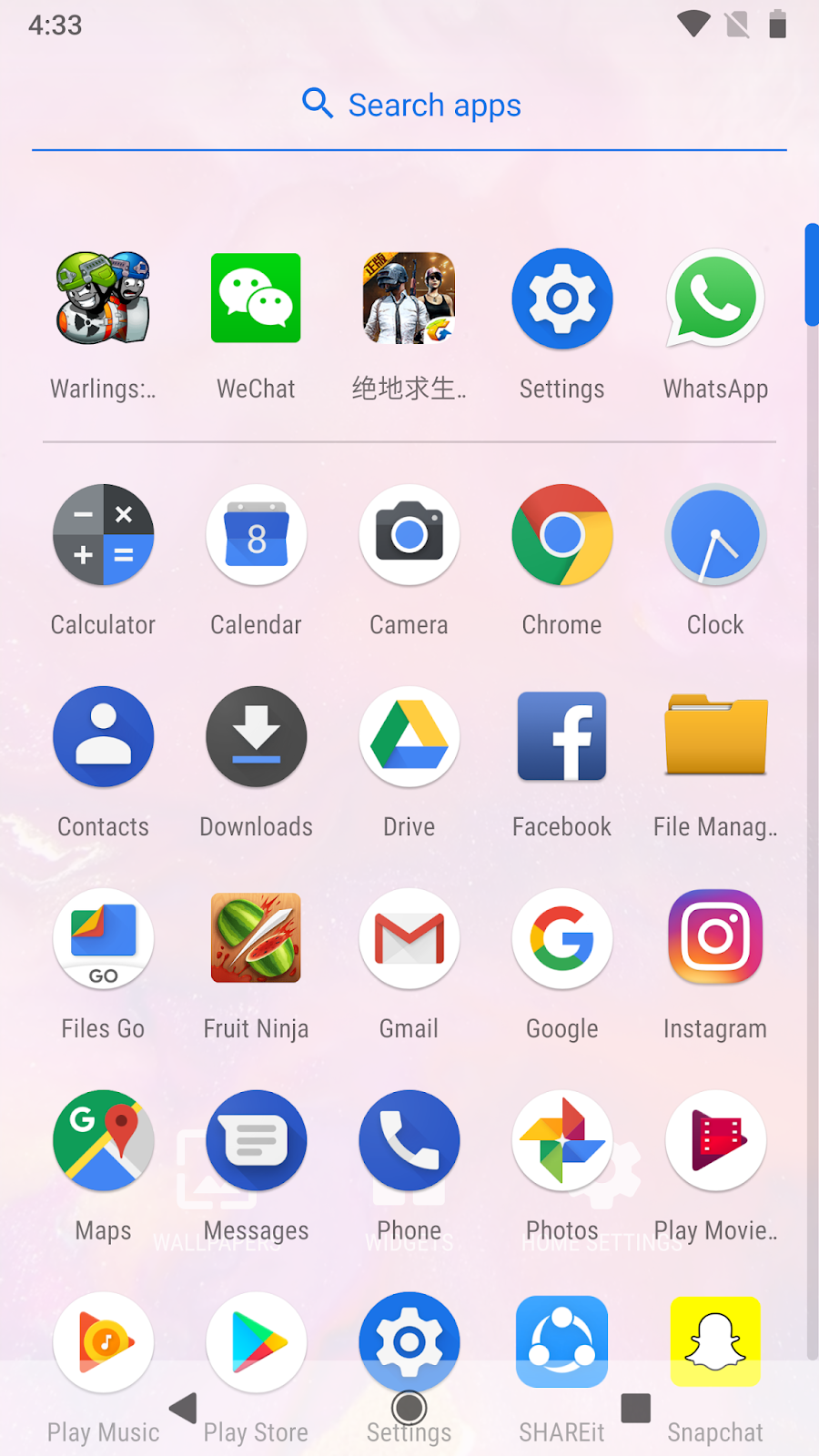The image showcases a smartphone screenshot set against a light pink background with the time displayed as 4:33 in the top left corner. The phone has full Wi-Fi connectivity and a battery level at approximately 75%. Below the status bar, there's a search bar featuring a magnifying glass icon and the text "Search apps" in blue, accompanied by a horizontal blue line beneath it.

The homescreen features six rows of five app icons each, organized in a grid layout. On the far right, there's a vertical blue scroll bar indicating the screen can be navigated further.

In the first row starting from the top left, the apps are as follows: "Warlings," "WeChat," an app with Chinese characters, "Settings," and "WhatsApp." The second row includes "Calculators," "Calendar," "Camera," "Chrome," and "Clock." The third row contains "Contacts," "Downloads," "Drive," "Facebook," and "File Manager." The fourth row lists "Files," "Go," "Fruit Ninja," "Gmail," and "Google." Finally, the fifth row from top to bottom includes "Instagram," "Maps," "Messages," "Phone," "Photos," and "Play Movies."

Each app icon is distinctly visible, creating an organized and easily navigable interface.